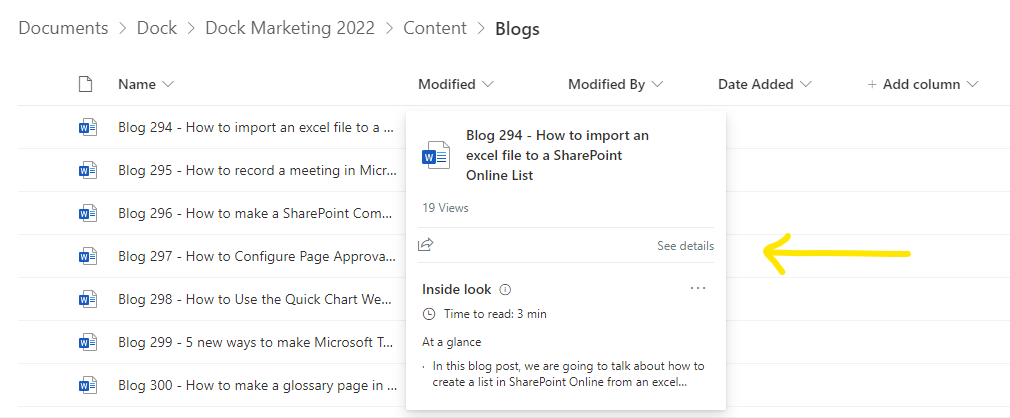### Blog Document Management Dashboard Screenshot

The screenshot displays a section of a computer application interface with a pure white background. 

**Header and Navigation:**
- At the top-left corner, there is a breadcrumb navigation path in grey text that reads: "Documents > Doc > Doc Marketing 2022 > Content > Blogs." The word "Blogs" is bolded to indicate the current folder.

**Column Titles:**
- Directly beneath the navigation path, several column titles are presented in bold text:
    - An icon of a piece of paper with the top-right corner folded.
    - "Name" with a downward-facing arrow indicating a sort option.
    - "Modified" followed by an arrow.
    - "Modified by" with an arrow beside it.
    - "Date added" followed by another arrow.
    - A light grey plus sign labeled "Add column."

**Document Rows:**
- Below the column headers, there are rows of document listings, each represented by an icon and a title:
    - The icon features a piece of paper with a folded top-right corner. There are blue lines and a blue square containing a white letter "W" on the left side, symbolizing the Word logo.
    - The document titles, listed vertically from top to bottom, are truncated as follows:
        1. Blog 294 - How to import an Excel file to a...
        2. Blog 295 - How to record a meeting in micro...
        3. Blog 296 - How to make a SharePoint com...
        4. Blog 297 - How to configure PageApprova...
        5. Blog 298 - How to use the QuickChart Wii...
        6. Blog 299 - Five new ways to make Microsoft T...
        7. Blog 300 - How to make a glossary page in...

**Document Detail Pane:**
- On the right side of the screenshot, there is a pop-up window displaying the details of one of the documents. This window provides additional information about the selected file, though the specific contents are not detailed in the description.